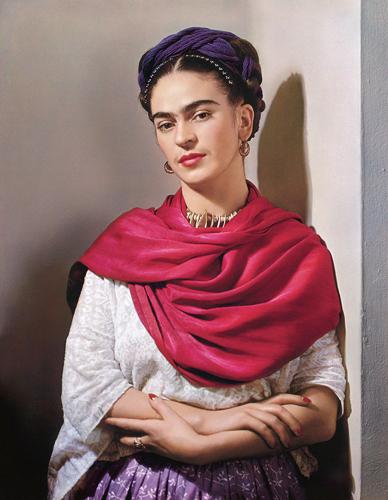In this picture, a woman is posed leaning against a wall, with the black shadow of her head visible on the surface behind her. Her hair is styled in an intricate braided updo, where two braids are crisscrossed around her head to form a headband effect. Interwoven through her hair is a strip of purple material, further accentuating the headband look. She is adorned with two large decorative hair combs on either side of her head, framing a central part in her hair.

The woman has brown eyebrows and wears vibrant red lipstick, and a delicate shadow of a slight mustache can be observed above her lip. Gold hoop earrings dangle from her ears, adding to her elegant appearance. Around her neck, she sports a choker-style necklace that appears to be made of shells.

Draped around her neck and over her shoulder is a piece of red cloth, contrasting with her white short-sleeve shirt. Her left middle finger is painted with red nail polish, and she wears a ring on her finger. Complementing her outfit is a purple skirt adorned with white flowers.